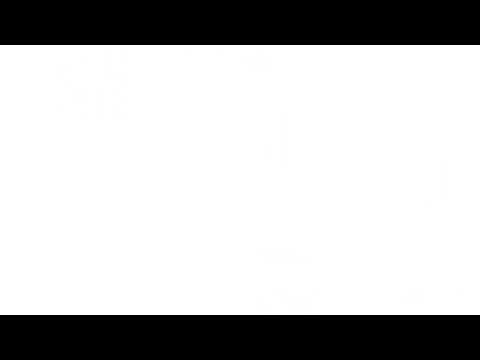The image is a vertically oriented, rectangular sign, consisting of a white space framed by two smooth, flat black stripes—one at the top and one at the bottom. Each black stripe spans the full width of the image and is about half an inch wide with pointed corners. The central area of the image is entirely blank, giving the appearance of an empty whiteboard or a wide-format video screen with unused white space between the stripes. The overall width of the image is a few inches, and the height of the white space in between the black stripes is approximately four inches.